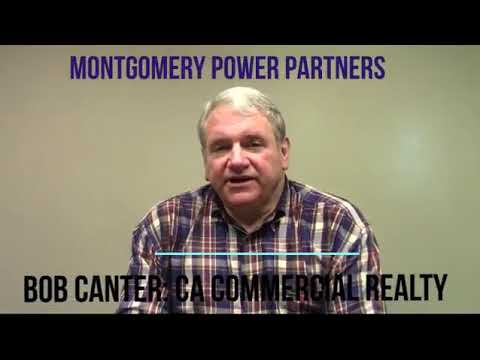The image shows an older white man, likely in his 50s or 60s, sitting and looking at the camera with his mouth slightly open. He has short gray hair and is wearing a flannel shirt adorned with a mix of red, blue, purple, white, and beige colors. The picture captures him from the stomach up, framing his shoulders and a bit of his arms. He is seated against a plain wall that appears brown-grayish or beige. At the top center of the screen, there is text in blue, all caps, reading "MONTGOMERY POWER PARTNERS". At the bottom, in black, all caps, it says "Bob Cantor: CA Commercial Realty," indicating that the image is likely part of a promotional advertisement for a realty company or realtor. Both texts are in a clear, easy-to-read font, possibly Arial. The overall look of the image suggests it's a screenshot from a social media platform like YouTube or Facebook.